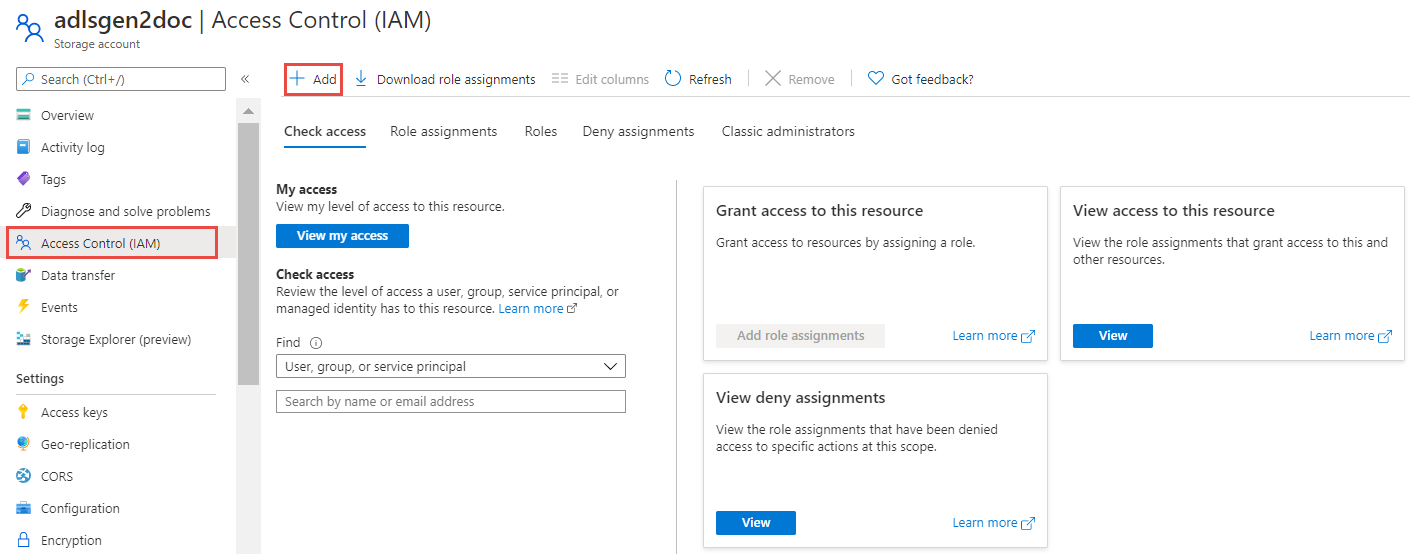The image features a white background with predominantly black text, resembling a screenshot from a computer interface. It lacks a distinct border, giving it an open, unframed appearance. At the top of the interface, the text reads "ADLS Gen 2 Dock" followed by "Access Control," indicating a section related to storage account management. Below this, a navigation menu includes entries such as "Overview," "Activity Log," "Tags," and "Diagnose and Solve Problems."

Highlighted with a red border, the "Access Control" section is clearly selected. Adjacent to this section, there's a menu featuring options like "Add" with a plus symbol, also marked with a red border, suggesting it has been clicked on. This part of the interface is dedicated to configuring access controls and permissions.

The headings in this area include "Check Access," "Role Assignments," "Roles," and "My Access." Under "My Access," the subtext reads, "View My Level of Access to This Resource," clarifying its function. Further to the right, another column displays functions like "Grant Access to This Resource" and a feature labeled "View Denny Assignments." 

In the upper right corner of the interface, there is an additional option titled "View Access to This Resource," encapsulating the various user permissions and roles configuration tools available in the interface.